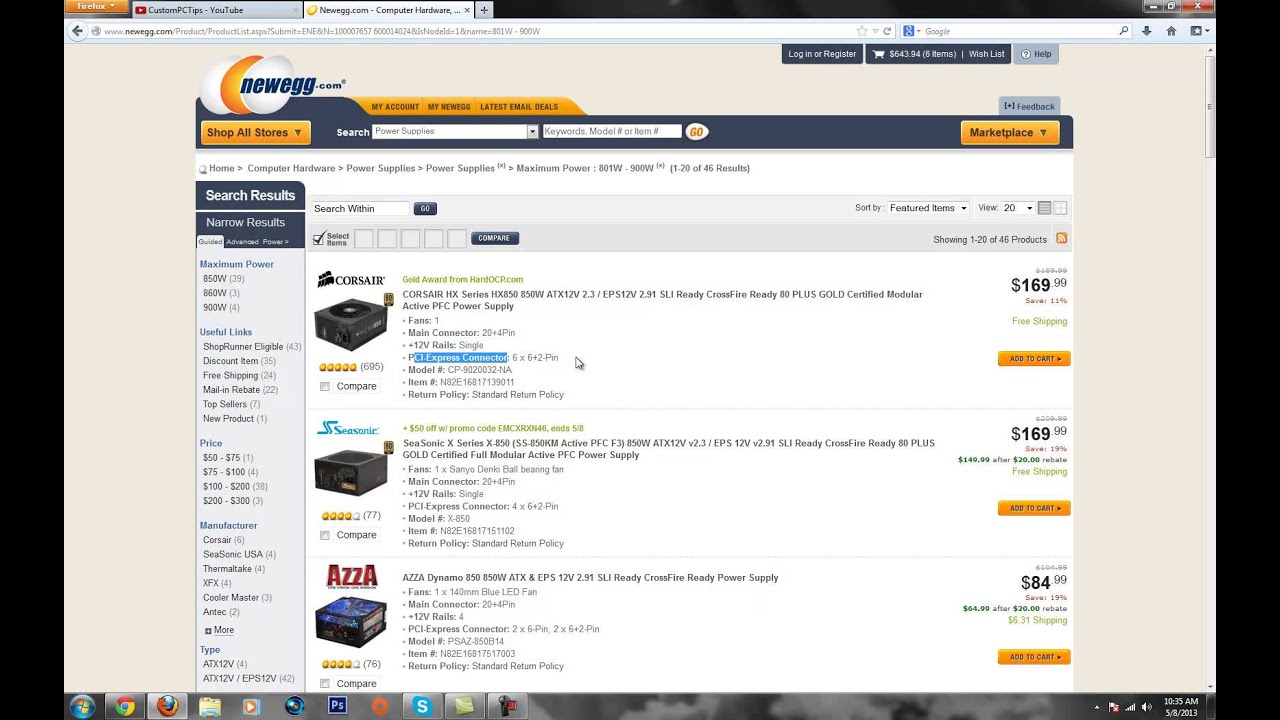The image is a screenshot of the Newegg website displayed on a Windows 7 computer, identifiable by its classic Windows 7 interface. The browsing is being done through a Firefox browser, which has two open tabs; one tab shows Newegg, while the other appears to feature a YouTube page, possibly titled "Custom PC Tips," although the exact text is not completely legible.

In the Newegg tab, the user has searched for power supplies. Several options are visible, with detailed listings for three power supplies specifically. The first two items are priced at $169.99 each, and the third one is listed at $85. These prices suggest that the power supplies are high-capacity units, likely intended for gaming or high-performance PCs. The page also includes various filters on the left side, enabling users to sort power supplies based on criteria such as price range, manufacturer, and maximum power capacity. This indicates that different PCs require different power outputs depending on their components and usage.

The website's main section features images of the power supplies, predominantly set against a white background, while a beige-colored frame surrounds the entire page, giving it a structured and neatly organized appearance.